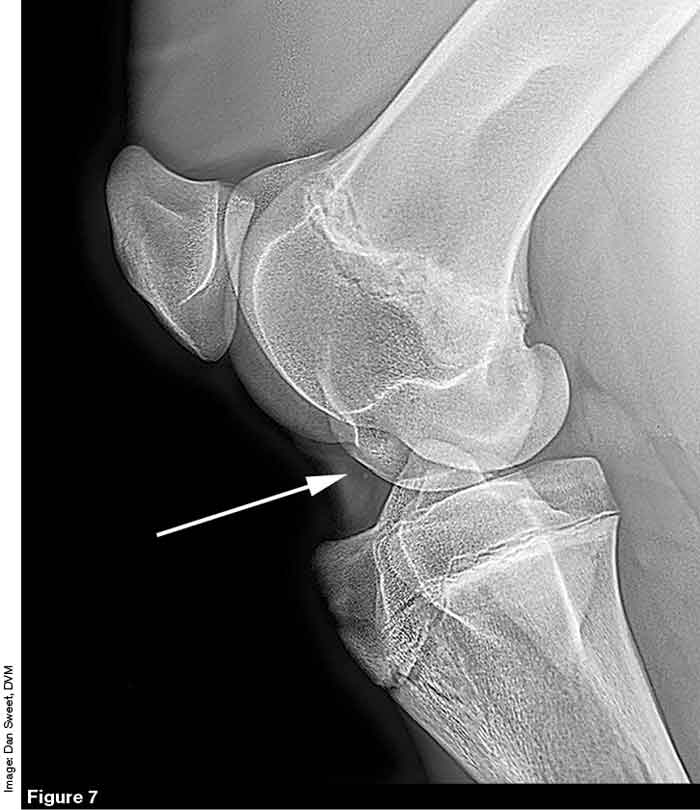The image is a detailed X-ray scan, likely intended for a medical textbook, as indicated by the caption "Figure 7" in white font at the bottom and image credit "Image Dan Sweet DVM" in small black font on the left. The scan depicts a close-up view of a human joint, displaying the black-and-white contrast typical of X-ray imagery. The X-ray captures three bones connected together—one large bone in the middle, another smaller bone slightly above it, and a third large bone at the bottom. There is a prominent white arrow pointing between the two larger bone segments, highlighting what appears to be a break, dislocation, or abnormality within the joint. The surrounding faint shadows hint at the presence of soft tissue, adding context to the bone structure and potential injury indicated by the arrow.